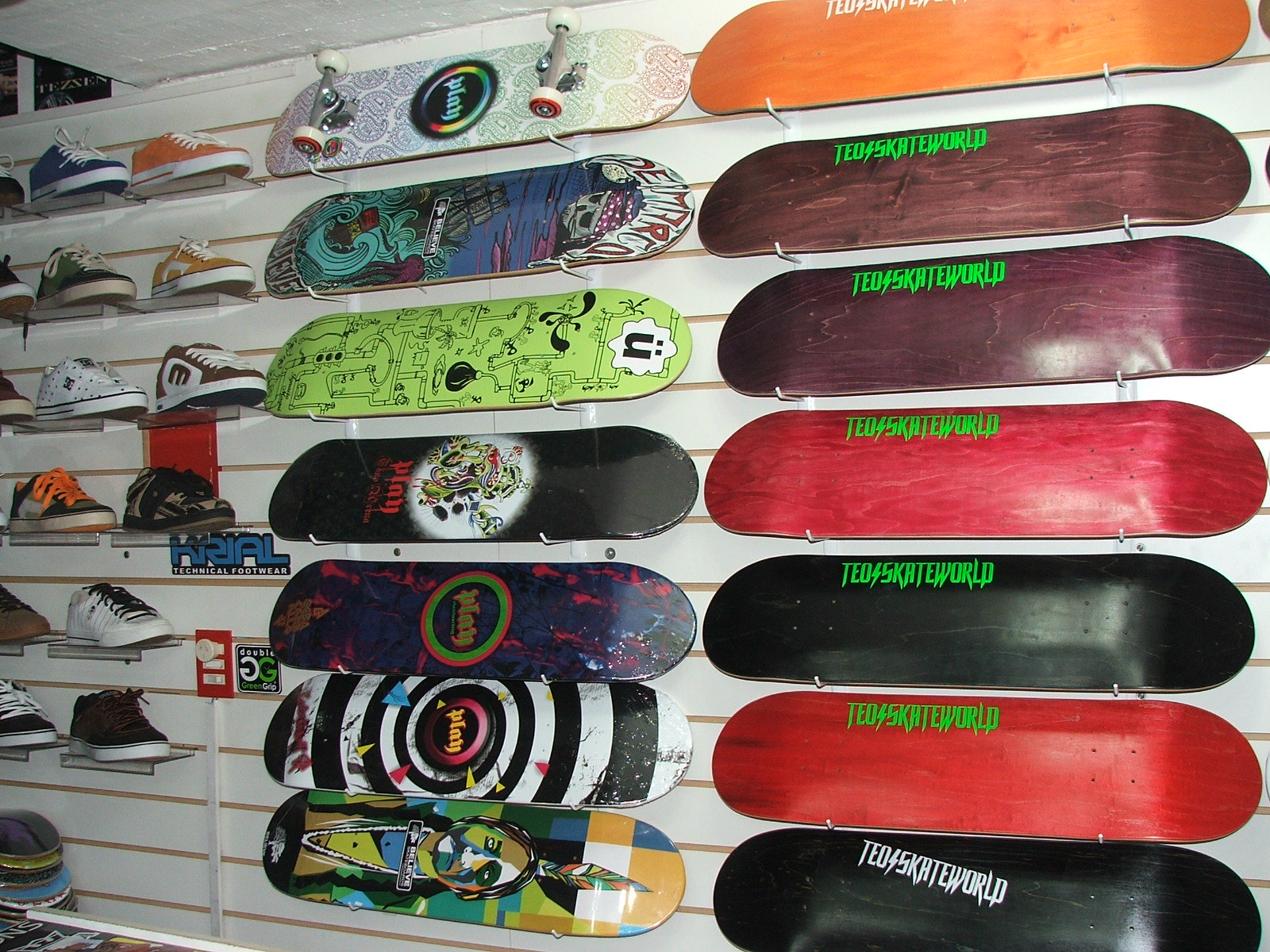This photograph captures a vibrant skate shop display. The focal point is an array of skateboard decks hung in neat rows on a white paneled wall with tan slits for shelf attachments. On the right side of the image, from floor to ceiling, are two columns of skateboards, mostly without wheels. The top left skateboard is the exception, featuring wheels. These decks predominantly have the logo "TEO Lightning Bolt Skate World" in neon green text, with variations in white. The colors of these boards range from black, red, and orange to different shades of purple. 

To the left of these branded decks, there is another set of skateboards featuring more intricate, colorful designs, including patterns, skulls, and hypnotic vortices. In the far left corner of the wall, there is a display of skateboard shoes, including brands like Converse, DC, Vans, and Etnies. The sneakers are organized on small plastic shelves and come in an array of colors and styles, from solid dark blue and orange to bold camouflage and polka dots. Each sneaker has white laces and flat bottoms, ideal for skating. Overall, the image showcases the eclectic and vibrant range of products typically found in a skate shop.